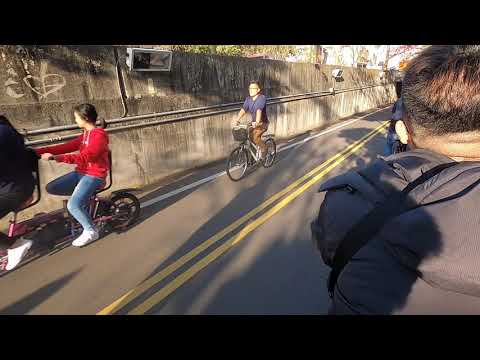The image depicts a narrow, horizontal bike trail marked by double yellow lines running down the center. On the left side of the path, bordered by a railing that overlooks a drop-off, possibly to railroad tracks or a river, there are two cyclists riding along. Nearby, three other cyclists are traveling in the opposite direction: two are stopped, peering over the railing, while a third rider is overtaking them. On the right side, partially cut off, is a man in a gray coat with a black strap, giving the impression of bicycling away. Behind him, a glimpse of another bike rider is visible. The detailed scene includes a man wearing tan pants and a gray shirt with a basket on his bicycle, and in front of him, a girl in a red hoodie with black hair riding a small bike. Another indistinct, dark figure rides further ahead. Surrounding the trail are trees, a cloudy sky, and possibly a rock face or additional structures that the onlookers might be examining. The path appears flanked by stone walls fitted with mounted lights, hinting at nighttime illumination. The scene is bordered in black at the top and bottom, framing the vivid activity within.